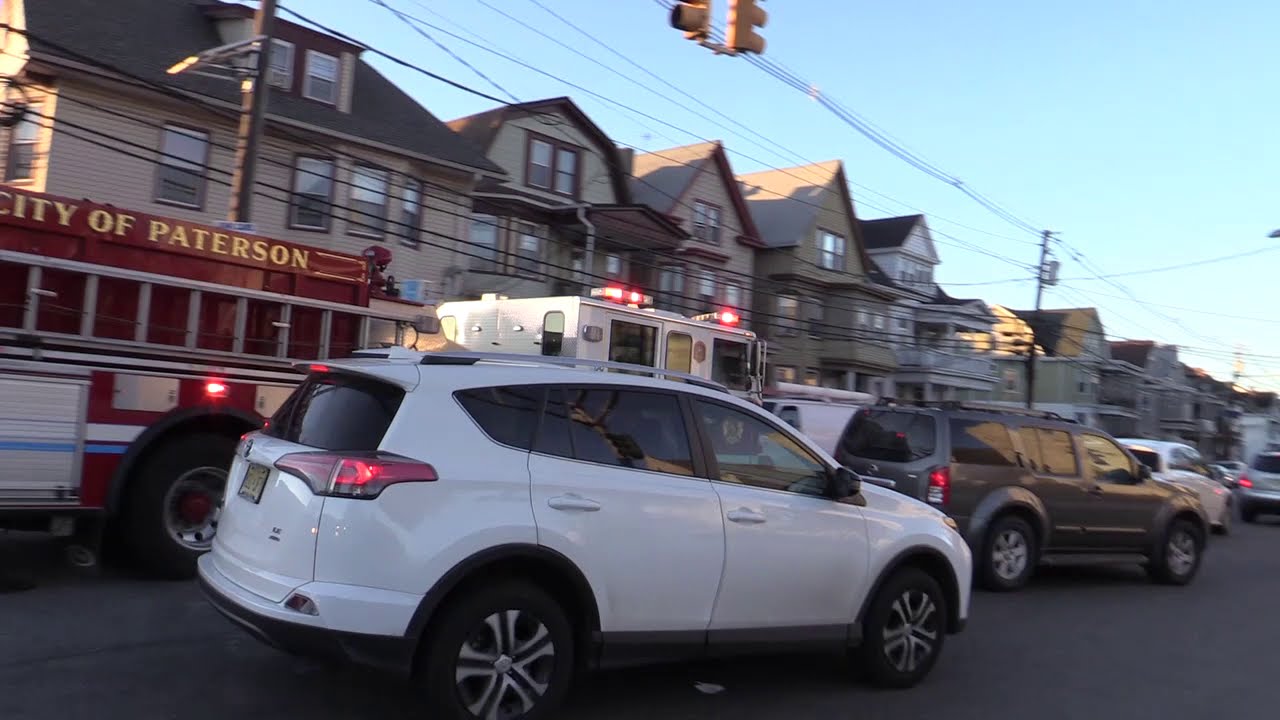The image depicts a bustling street scene under a clear, blue daytime sky. Dominating the center foreground is a white SUV with black tires and tinted windows, positioned directly behind a dark gray SUV. Further back, a red and white fire truck, distinguished by its flashing lights and "City of Paterson" signage atop a ladder, is seen approaching from the left. Surrounding these vehicles are additional cars along a gray roadway. The middle top of the image features a yellow traffic light, while utility poles and power lines stretch across the scene. The background displays a closely-packed row of neutral-toned row houses or townhouses with windows, blending yellow, gray, and brown hues. The scene showcases the intricate details of an urban environment, underscored by clear blue skies and typical city infrastructure.